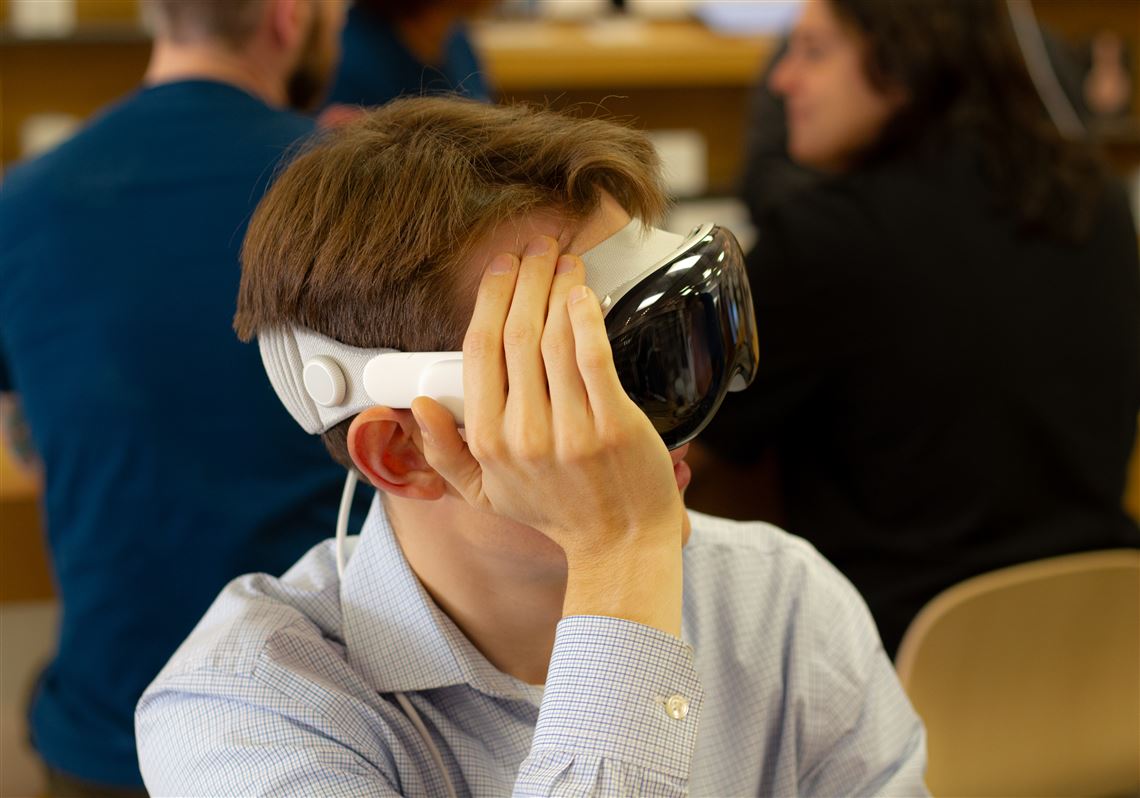This detailed close-up photograph features a young man, possibly a teenager, wearing a bulky, futuristic VR headset. The headset, which is primarily white and wraps securely around his head, includes a thick black lens piece at the front with lenses that cover both eyes. The white band, made of a durable and expandable material, ensures the device is firmly in place. The young man is dressed in a white checkered collared button-down shirt, with his short-cropped brown hair visible above the headset. His right arm is folded at the elbow, and his hand is grasping the side of the VR device, presumably adjusting or supporting it. His skin is white, and he is seated next to a tan chair. In the blurred background, two additional individuals, a man on the left and a woman on the right, are seated at a table with a counter behind them. The young man appears to be gazing off to the side through the intriguing black lenses.